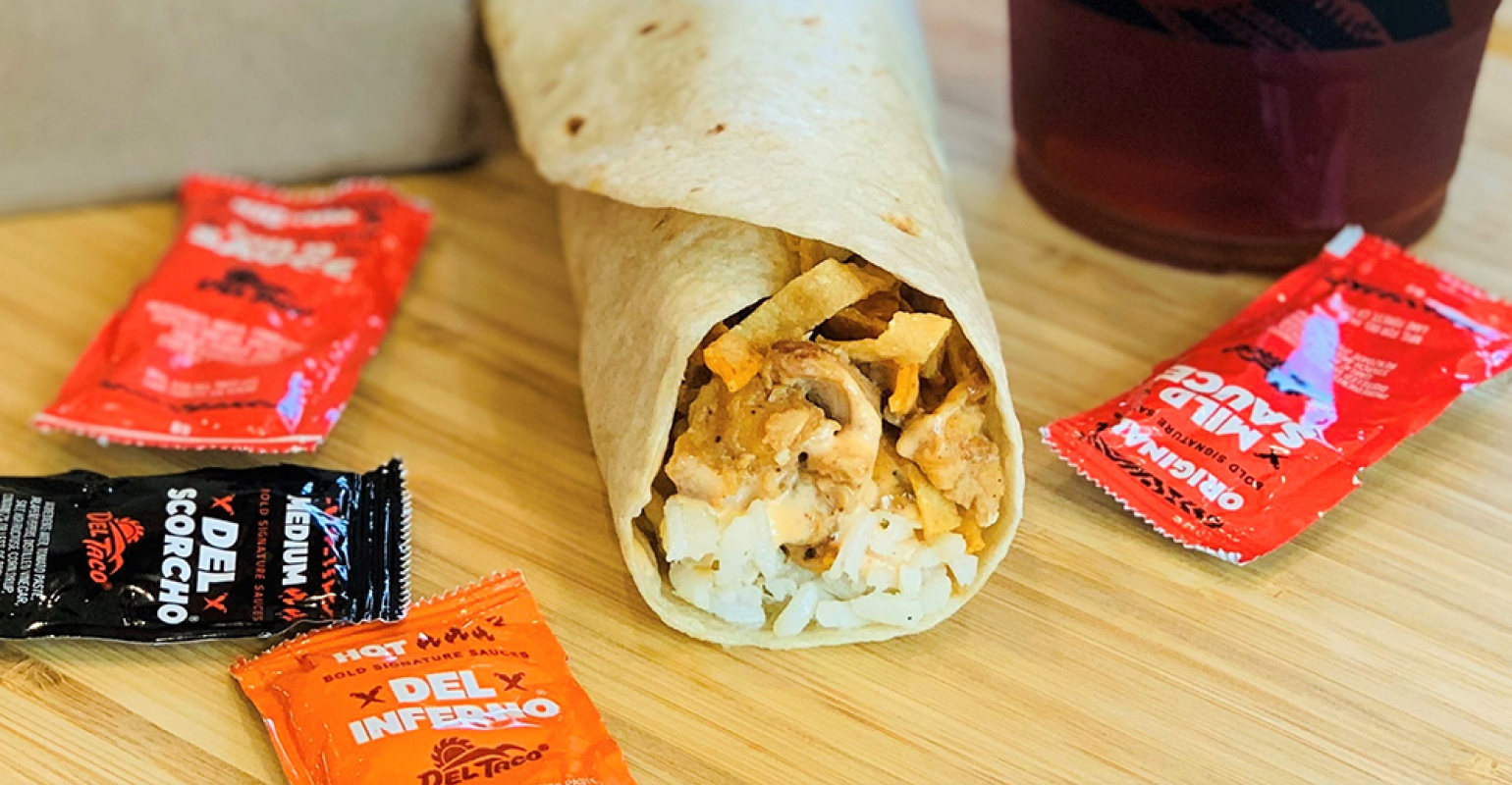The photograph depicts a small Mexican burrito from Del Taco, carefully placed on a wooden tabletop. The burrito is wrapped in a soft flour tortilla and filled with rice at the bottom, a modest amount of chicken at the center, and topped with crispy tortilla strips. Surrounding the burrito are various hot sauce packets, including a red packet labeled "mild salsa," an orange packet marked "Del Inferno" indicating its hot spiciness, and a black packet branded "Del Scorcho." Additionally, the Del Taco logo is visible on one of the sauce packets. In the bottom portion of the image, there's a glimpse of a glass containing a dark liquid, further enhancing the setting's casual dining atmosphere.